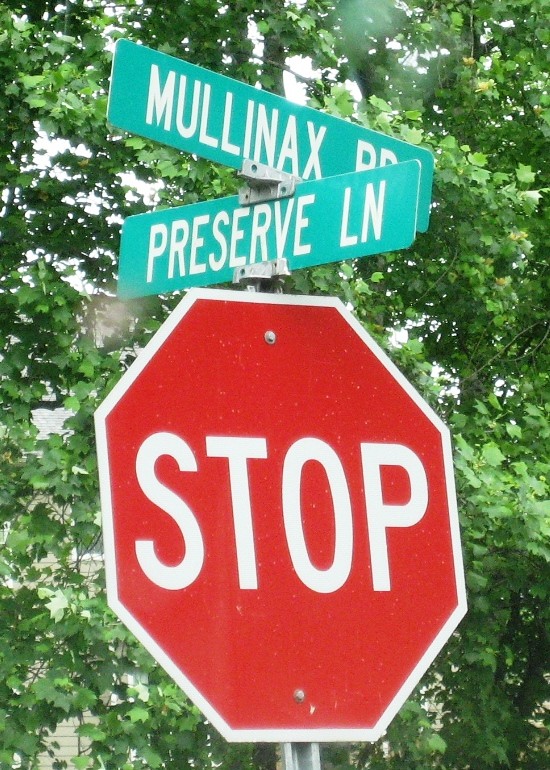The photograph captures a sunny daytime scene featuring a traditional hexagonal stop sign with a red background and white "STOP" letters, outlined in white and riveted to a steel pole. Above the stop sign, there are two green road signs with white text, also affixed with silver rivets. The top road sign is slightly angled to the right and reads "MULLINAX ROAD," while the one below is angled to the left and says "PRESERVE LANE." Both road signs are rectangular in shape. In the background, a lush canopy of green trees and vines can be seen, with sunlight filtering through the leaves. Additionally, there is a faint outline of a building with a gray roof visible in the distance.